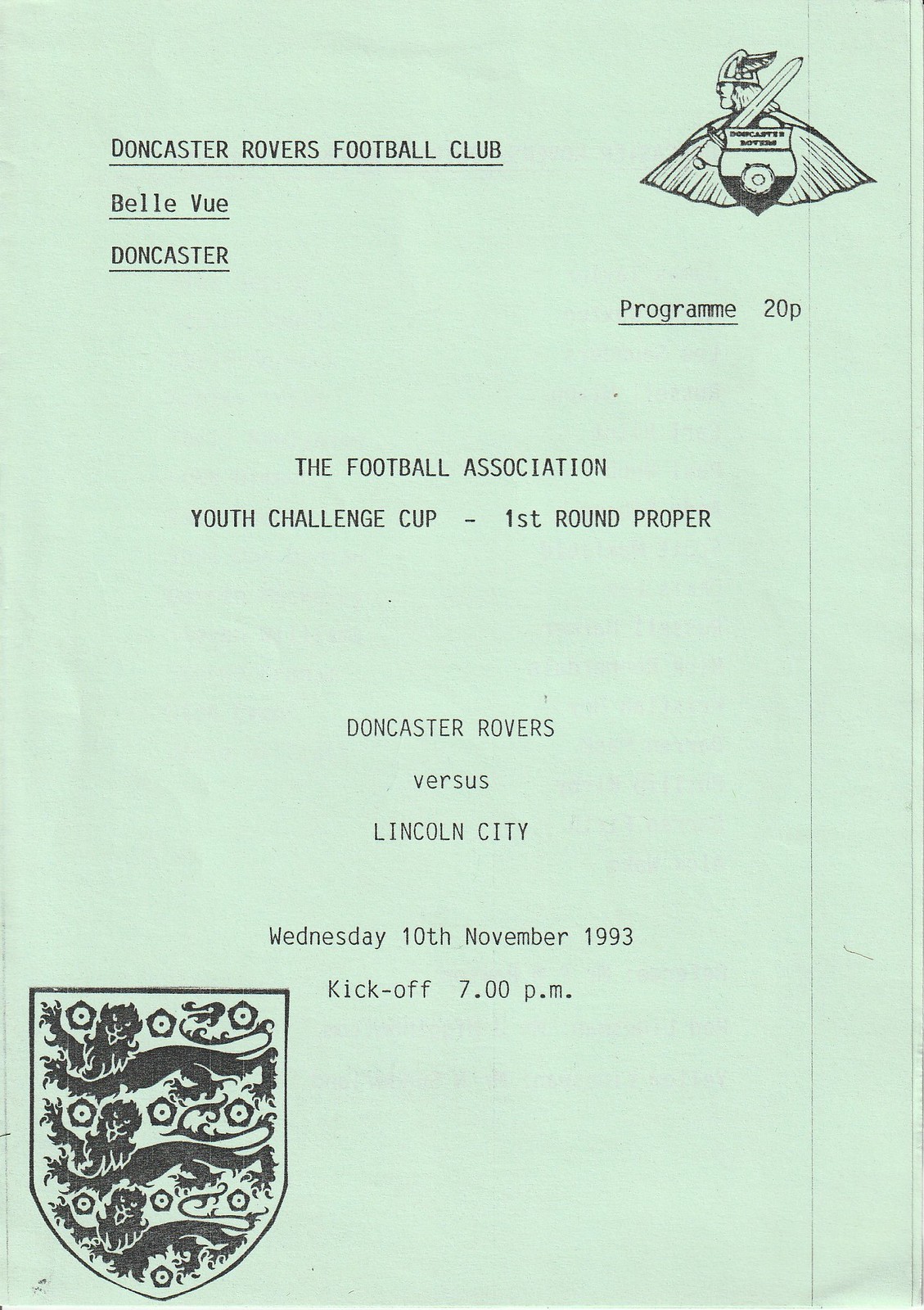This image is the front cover of a program or magazine for a soccer game, specifically the Football Association Youth Challenge Cup First Round Proper, featuring a match between Doncaster Rovers versus Lincoln City. The program, priced at 20p, is printed with black ink on a light green, soft-colored paper. At the very top, it reads "Doncaster Rovers Football Club, Bellevue, Doncaster." On the top right corner, there is an emblem depicting a Viking with a sword, a cape, and a shield, and directly beneath it, the price "Program 20p" is noted. On the bottom left corner, there is a coat of arms logo. Central to the cover is the key event information: "The Football Association Youth Challenge Cup First Round Proper." Further down, it details the match specifics: "Doncaster Rovers versus Lincoln City, Wednesday, 10th November 1993, kickoff 7 p.m." The design and layout suggest it is an official program typically provided to attendees of the soccer game.